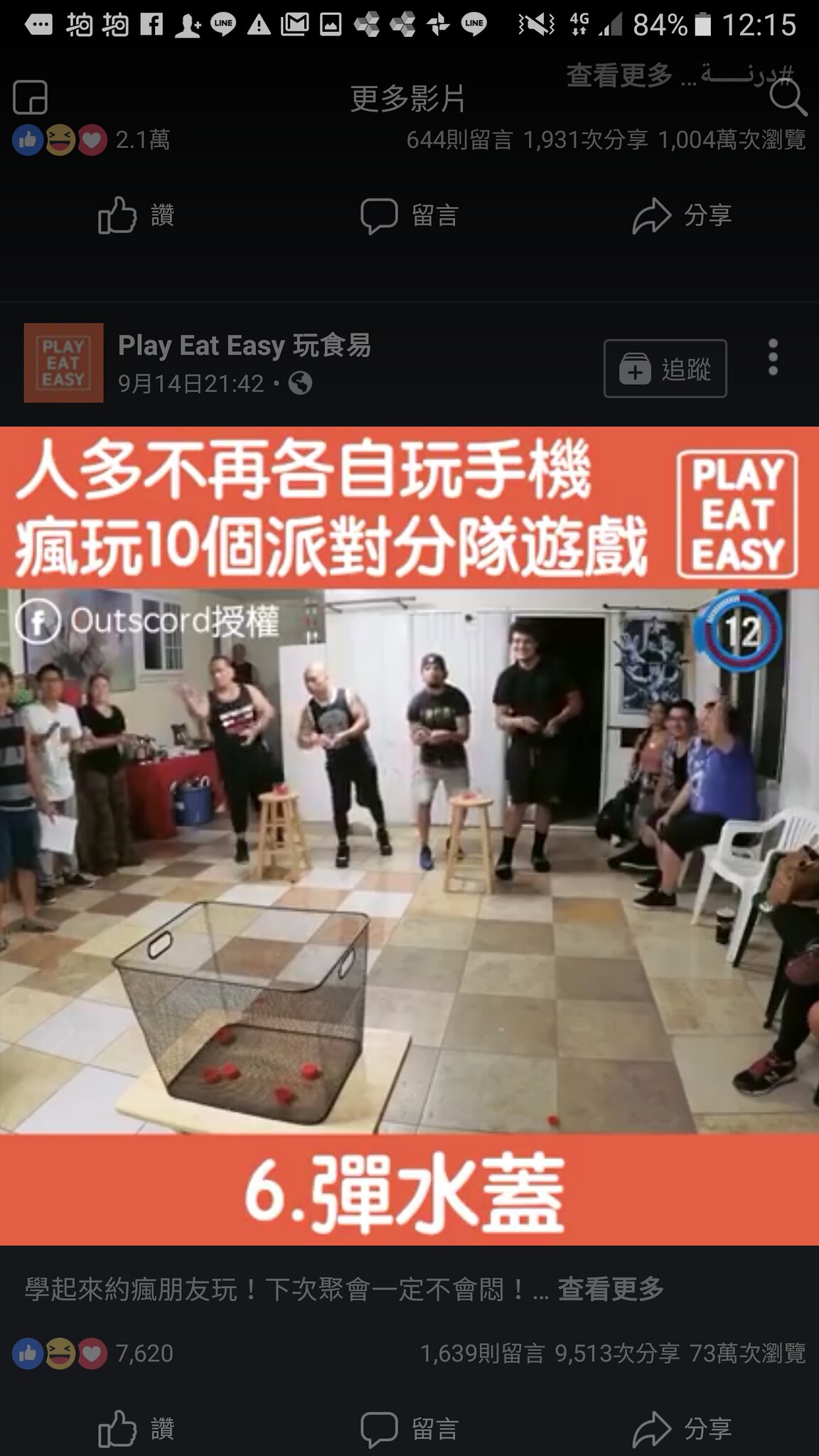This image appears to be a screenshot from a cell phone, capturing a social media post or advertisement. At the top of the screen, there is a timestamp reading 12:15, an 84% battery indicator, a 4G logo, and various app icons such as Gmail and Facebook, suggesting it is taken from a smartphone. The post prominently features the text "PlayEatEasy" against an orange background with the phone number 914-2142 in white print. Additionally, there is a Facebook icon accompanied by the word "outscored".

In the image itself, there are a group of people inside a room with a brown, checkered tile floor. Four men are engaged in a game involving throwing balls into a plastic tub or glass box that sits atop a tray table in the center of the room. The game appears to have elements of skill, as there are several objects inside the tub suggesting previous successful throws. The scene is watched by other individuals either standing or sitting off to the sides. The room also features some Asian text, which contributes to an overall East Asian aesthetic and context.